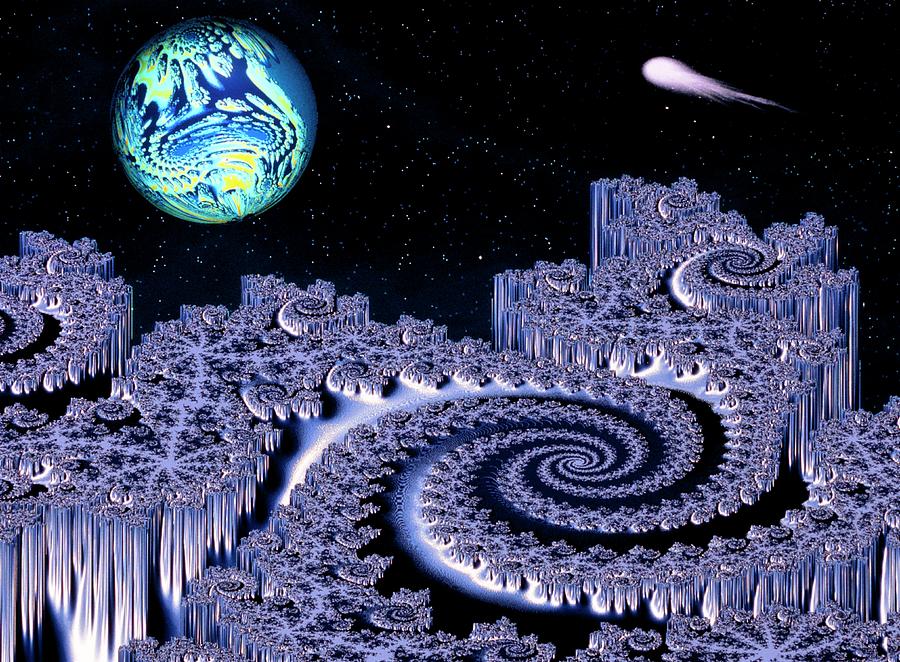The image is an intricate piece of science fiction art set in outer space, showcasing a mesmerizing, trippy space-oriented fractal scene. Against a black, star-filled background, a vibrant planet floats in the top left corner, radiating hues of blue, green, aquamarine, and yellow. In the top right, a dynamic comet shoots upward, with a vivid purple and white trail streaming behind it. Dominating the foreground, a breathtaking cliff-like structure composed entirely of metallic, ice-like fractals and spirals extends downward into a three-dimensional form. This complex fractal, rendered in shades of blue, white, black, and purple, repeats and intertwines, creating an intricate, otherworldly landscape that captures the imagination.